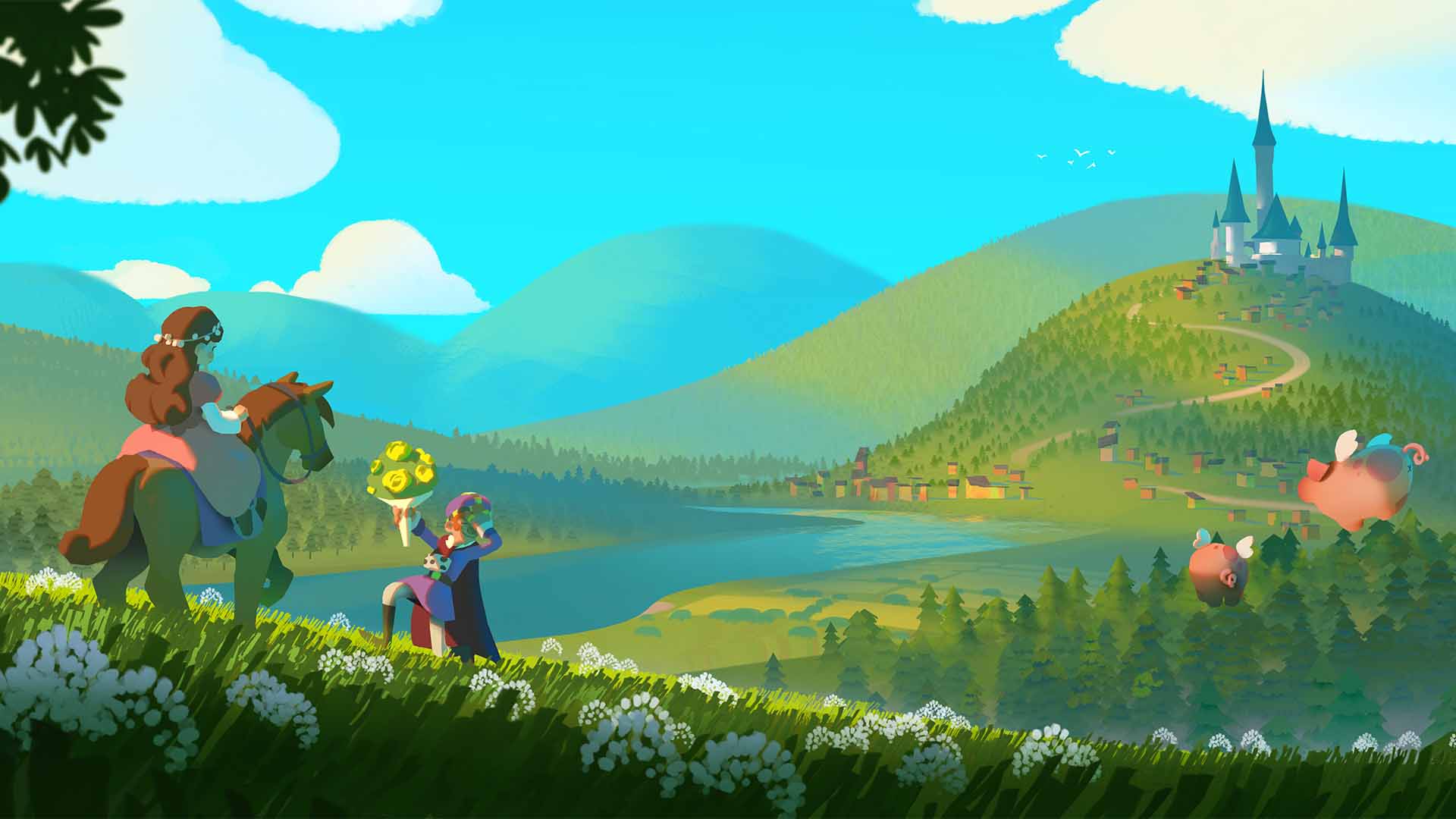In a vibrant, cartoonish illustration, a whimsical scene unfolds in a lush green field leading up to a classic fantasy castle with tall cylindrical towers and conical rooftops. The bright blue sky is dotted with fluffy, bubbly clouds. In the foreground, a maiden with long brown flowing hair adorned with a white floral crown rides a green horse with a brown mane and tail. She wears a pink dress, adding a touch of elegance to her serene presence.

Kneeling in front of her, a gentleman draped in a cape offers a bouquet of yellow flowers, his arm extended upward in a gesture of devotion. The scene is further enriched by the presence of flying pigs with wings on the right side, adding an element of playful fantasy.

The field is speckled with white flowers and green grass, while the landscape features rolling hills dotted with pine trees. A winding pathway ascends one of the hills, leading to the majestic castle. Below the hill, a river meanders through the scene, and a cluster of houses, likely belonging to villagers, can be seen. The overall composition captures a moment of romantic chivalry in an enchanting fairytale setting.